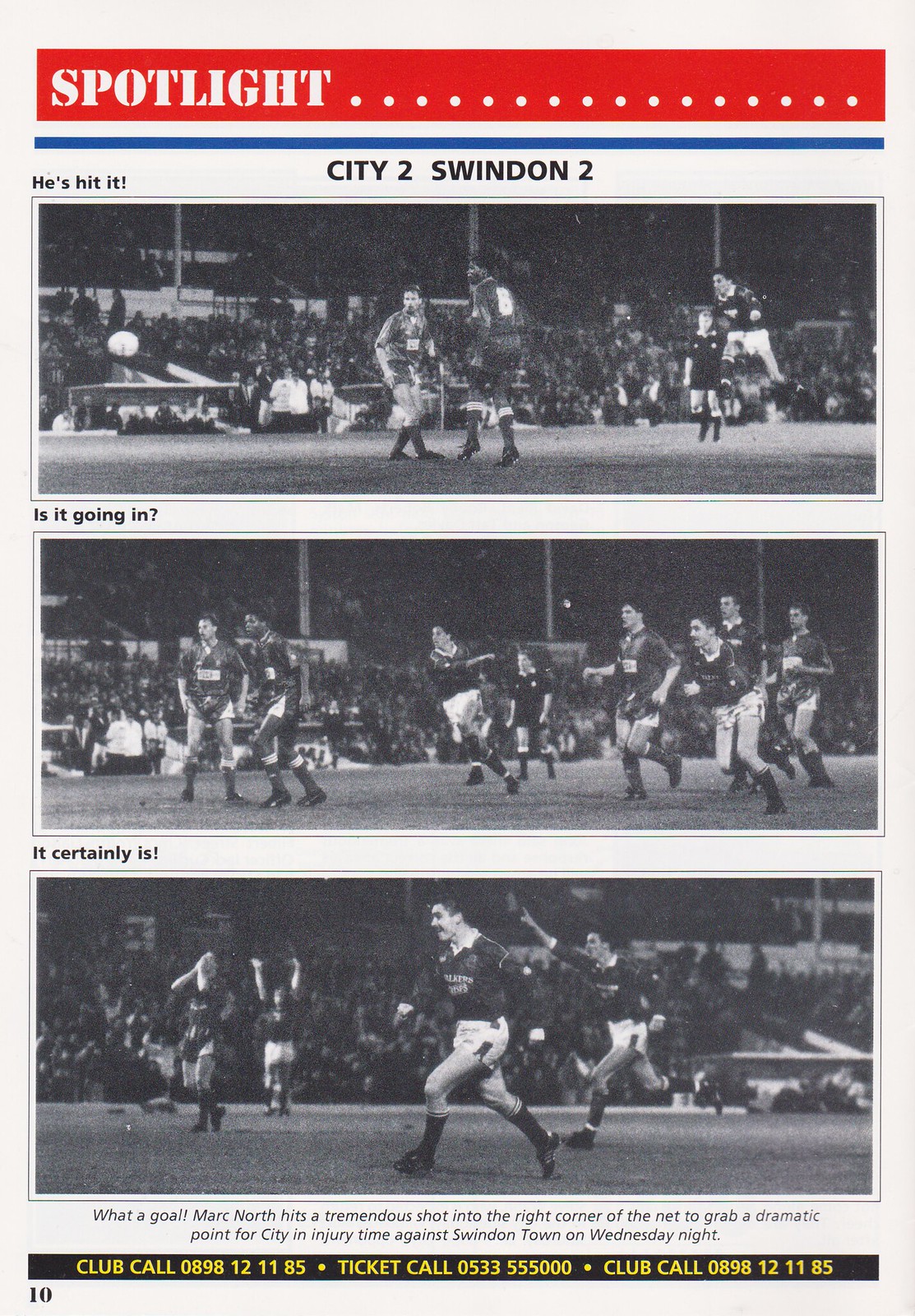The image is a vintage newspaper clipping or a page from an old sports magazine, likely from the 1960s or 1970s. At the top of the page, "Spotlight" is prominently written in white text on a red ribbon background. Below this header, the score "City 2, Swindon 2" is displayed.

The main content features a sequence of three black-and-white photographs documenting key moments of a soccer game. The first image, accompanied by the caption "He's hit it," shows a player making a shot. The second image, labeled "Is it going in?" captures the ball mid-air as players and the crowd watch intently. The third photo, captioned "It certainly is," depicts the moment the ball hits the back of the net, and a player is seen celebrating.

At the bottom of the page is a detailed description: "What a goal! Mark North hits a tremendous shot into the right corner of the net to grab a dramatic point for City in injury time against Swindon Town on Wednesday night." Additional information for the club, including a "club call" number and a "ticket call" number, is also present at the bottom of the page. The overall aesthetic, with its tan, red, white, blue, black, and various shades of gray, evokes a nostalgic feel of a bygone sports era.